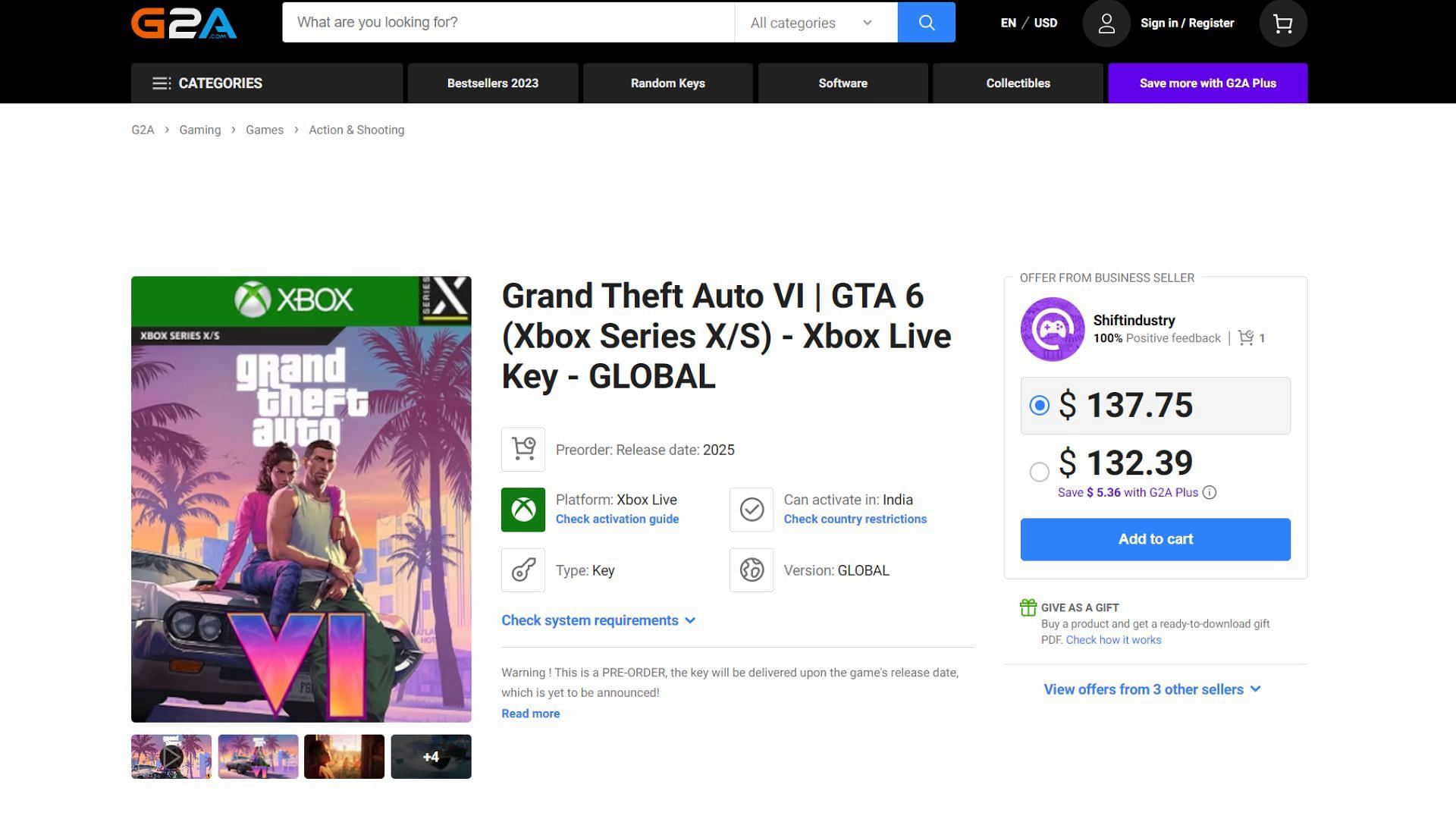This image captures the Grand Theft Auto (GTA) section on the G2A website. The website features a sleek black background header where the G2A logo is prominently displayed—'G' in orange, '2' in white, and 'A' in blue. To the right, there is a white search bar with placeholder text, "What are you looking for?" followed by a dropdown menu labeled "All Categories." Adjacent to the search bar, a blue search button with a white magnifying glass icon is visible. Further to the right, there are options to sign in, register, and view the shopping cart.

Beneath the G2A logo, there are several categories listed horizontally: Bestsellers, Random Keys, Software, Collectibles, and a promotional link "See more with G2A Plus."

In the lower section, against a white background, the cover art for the Grand Theft Auto 6 (GTA 6) Xbox edition is featured. The cover has the characteristic green Xbox branding at the top. To the right of this cover image, the game is described in detail: "Grand Theft Auto 6 (GTA 6) Xbox Series X/S, Xbox Live Key, Global." The price is listed as $137.75 or a discounted price of $132.39. Below the price, there's a blue "Add to Cart" button.